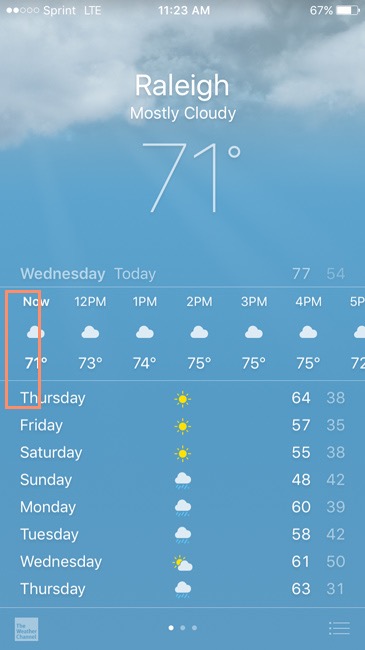This is a detailed screenshot from a weather app displayed on a mobile phone, featuring a background that mimics a blue sky with a few clouds at the top. The upper section of the screenshot contains status information about the phone in white font, including two white dots followed by three empty dots, "Sprint LTE," the time "11:23 AM," the battery percentage "67%," and a battery icon. Below this status bar, against the cloudy sky background, the text reads "Rally, Mostly Cloudy, 71°" in white font. 

Further down, it shows "Wednesday, Today, 77 / 54," indicating the high and low temperatures for the day. Below this, there's an hourly forecast section. A red vertical rectangle highlights the "Now" time slot, which shows a cloudy icon and a temperature of 71°. The subsequent hourly forecasts are as follows: at 12 PM, the temperature will be 73°; at 1 PM, 74°; at 2 PM, 75°; at 3 PM, 75°; at 4 PM, 75°; and at 5 PM, 72°. 

The bottom part of the screenshot displays a five-day forecast:
- Thursday: High of 64°, Low of 38°
- Friday: High of 57°, Low of 35°
- Saturday: High of 55°, Low of 38°
- Sunday: High of 48°, Low of 42°